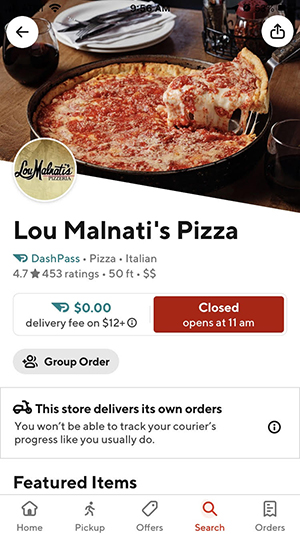Here is the cleaned-up and detailed caption for the image described:

---

This is a screenshot from a food delivery app on a smartphone. At the top of the screen, there's a picture of a deep-dish pizza with a golden-brown crust. A utensil is pulling out a gooey, cheese-laden slice from the pan. The pizza is set on a wooden table, surrounding it are a stack of white plates, utensils, napkins, and a glass of red wine.

In the upper section of the app, there's a circular logo that reads "Lou Malnati's, Pizzeria." Below the logo, the title "Lou Malnati's Pizza" is prominently displayed alongside indicators showing that it offers DashPass, is categorized under Pizza and Italian cuisine, has a 4.7-star rating based on 453 reviews, is located 50 feet away, and the pricing is denoted by two dollar signs ($$).

Further down, it states that the delivery fee on orders $12 and over is $0.00. Next to this information, there is a red button that indicates the restaurant is currently closed and will open at 11 a.m. Beneath this button, there is a rectangular button labeled "Group Order" with an icon of a person and the shadow of another person behind it.

A notification below this button informs users that "This store delivers its own orders. You won't be able to track your courier's progress like you usually do," accompanied by a graphic of a scooter. The section is followed by a list titled "Featured Items," and at the bottom of the screen, there are navigation tabs labeled Home, Pickup, Offers, Search, and Orders.

---

This caption provides a comprehensive and organized description of the screenshot.